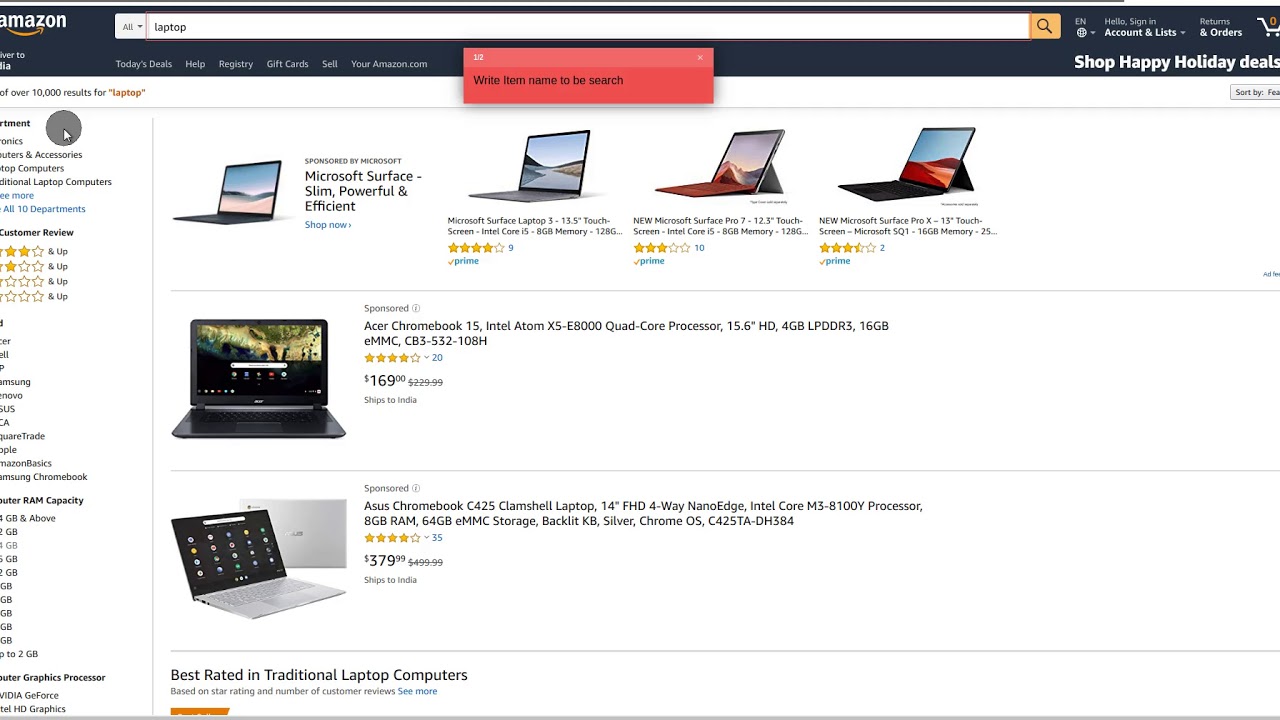A detailed screenshot of the Amazon website is displayed, showcasing a search for "laptop" in the search box. Below the search box are various search results. Notably, there is a small pop-up window in the upper part of the page, marked with "1/2" and an 'X' to close it in the upper right corner. This pop-up includes a text field for specifying the item name to search, with a typical mouse cursor highlighted inside a gray circle indicating its location.

The screen is formatted with Amazon's customary header at the top. On the left-hand side, various filter options are available to refine the search results. To the right, the main content area displays four rows of laptop listings, with the bottom row partly visible.

The first row features sponsored laptops, including a generic ad sponsored by Microsoft, showing an image and a "Shop Now" button. To the right, there are three specific laptop listings. The second and third rows also present sponsored laptops, showcasing products from brands like Acer and Asus. The final row, labeled "Best Rated Traditional Laptop Computers," is partially truncated.

Additional information includes a mention of a book by writer Mary Sandy, a resource recommended for students seeking laptops.